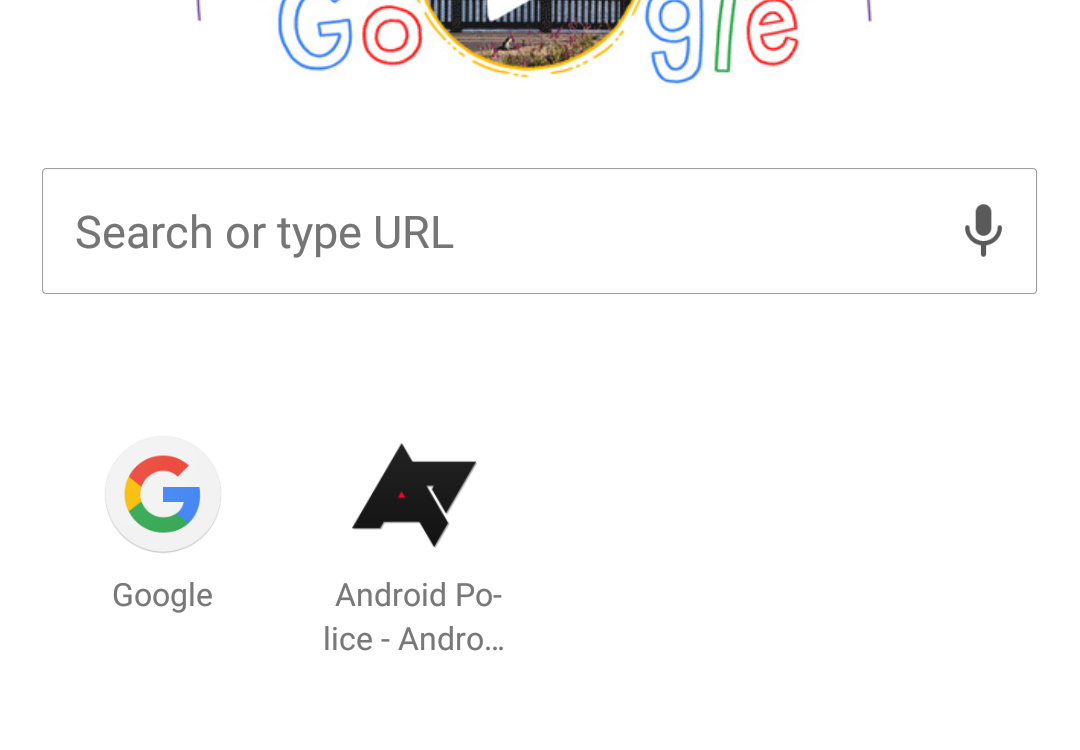This image depicts a cropped view of the Google homepage on a mobile device. The focal point is a special Google Doodle, featuring the company's logo redesigned with unique artistic elements. The traditional blue capital "G" is followed by a lowercase red "o." The second "o" is replaced by an ornate picture frame with a yellow-gold border showcasing an illustration of rails and flowers. This graphic element contains a partially visible white play button. To the right of the illustration, the logo continues with a lowercase blue "g," a green "l," and a red "e." Beneath the logo, there is a search bar that prompts users to "Search or type URL," accompanied by a microphone icon for voice input. Additionally, there are shortcuts below the search bar, including the Google "G" symbol inside a white circle and a link labeled "Android Police," indicating frequently visited pages for quick access.